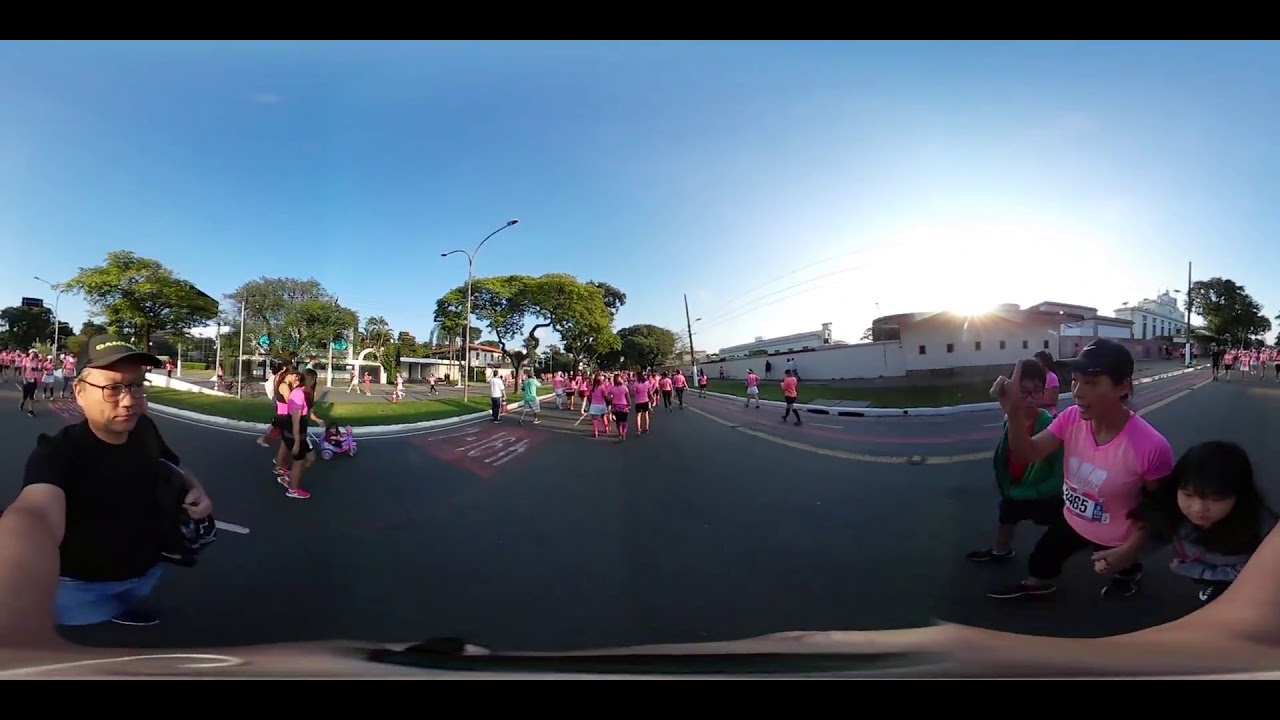This image captures a vibrant and bustling charity event, likely a breast cancer awareness marathon or walk, taking place on a busy, curving road. The participants, predominantly dressed in pink shirts, flood the center lane and stretch into the background, underlining the large scale of the event. In the foreground, a man in a pink shirt is seen taking a picture next to a child and another man. On the left side of the image, another man in a black shirt, black cap, and blue shorts stands observing the scene. Notably, a woman with her hand on the hood of a car can be seen, presumably guiding the vehicle to avoid stepping on walkers. 

The backdrop includes a prominent white building with green lawns and hedges, distinctive with its arches on the far right, suggesting a government or institutional edifice. On the left side, a park area with various individuals walking or standing adds to the communal feel of the event. This well-attended gathering clearly reflects its purpose: to raise awareness and funds for breast cancer, demonstrating community solidarity and support.